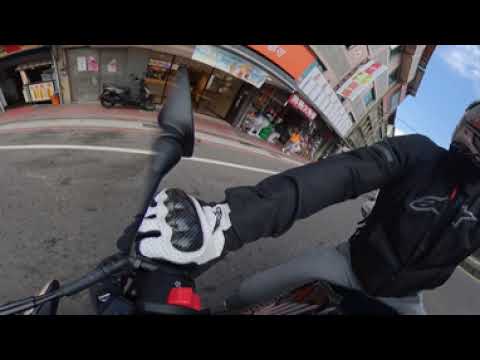This photograph, captured with a fish-eye lens from the perspective of the motorcycle handlebars, shows a motorcyclist navigating a city street, likely in an Asian city or Chinatown, deduced from the Chinese lettering on the buildings. The motorcyclist is partially visible on the right side of the image, sporting a black helmet, a black riding jacket, and white and black gloves, with a firm grasp on the left handlebar that features a prominent red button. He's clad in light-colored (likely gray) jeans. The warped, curvy image emphasizes his gloved hand, the handlebar, and a black mirror. The backdrop reveals a multi-story streetscape with shops on the ground floor and potential living quarters above, connected by a pinkish-red sidewalk. The street itself is a regular paved road, possibly with a bicycle lane, and the photo also includes a glimpse of another motorcycle and a pedestrian in yellow. The sky is a clear blue, visible in the upper right corner of the frame, adding vibrancy to the urban scene.